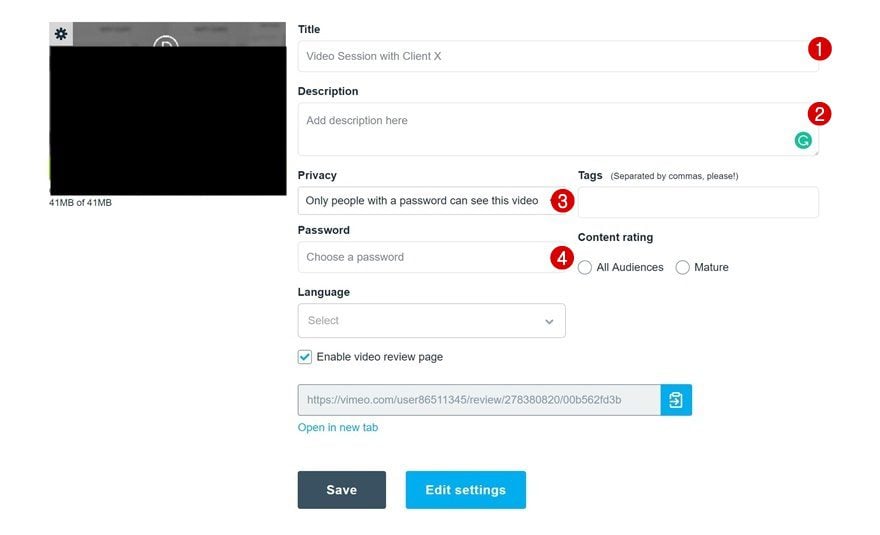This image depicts the interface of a video upload platform, reminiscent of popular sites such as Vimeo or YouTube. Prominently displayed are fields designated for entering the video's title and description, which are currently devoid of any content, suggesting this is a tutorial or instructional guide. The tutorial is likely designed to familiarize users with the process of uploading videos. Additionally, the image highlights various settings options available for customization, with a distinctive blue button specifically for accessing the settings menu.